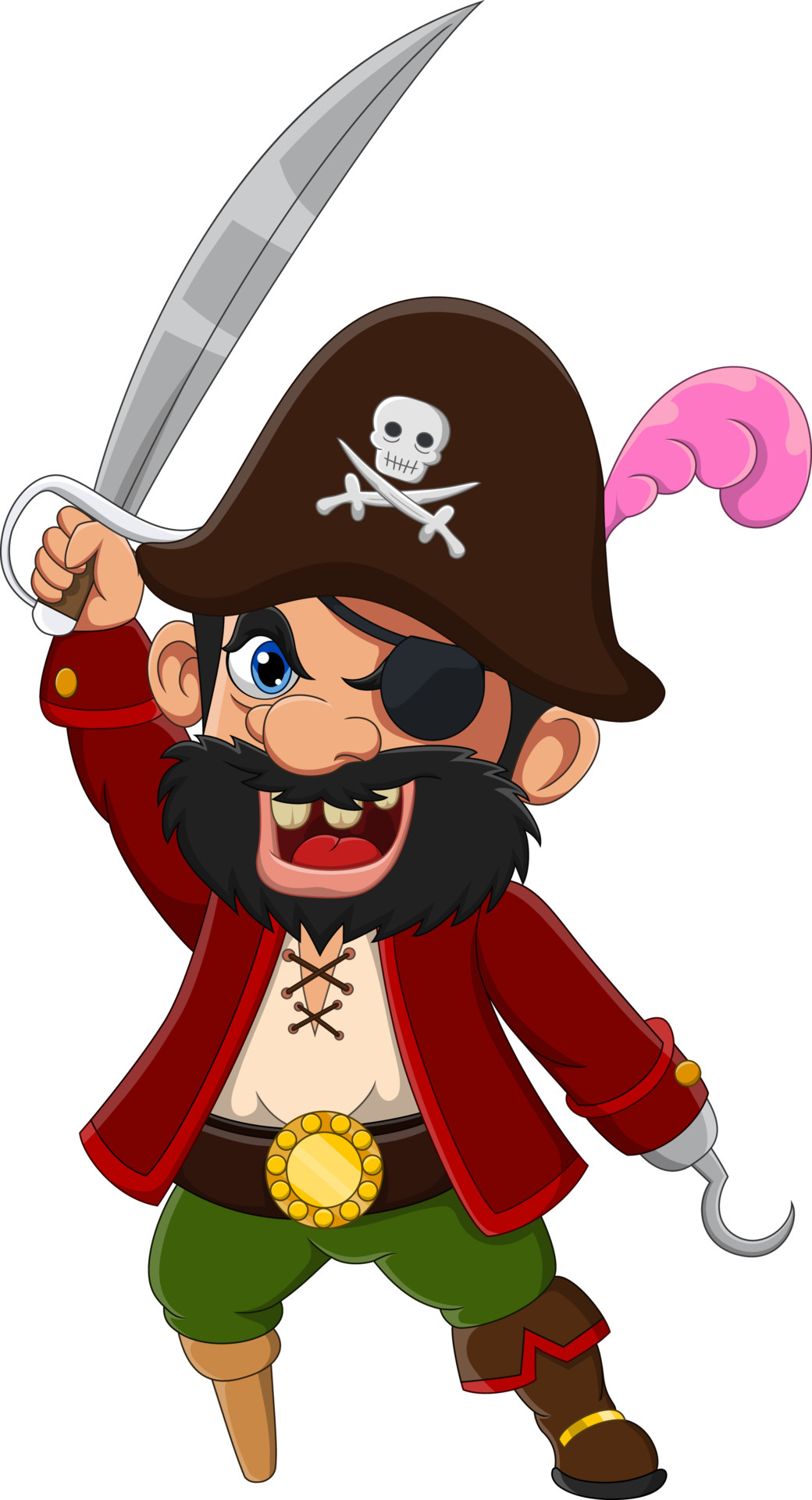This detailed image depicts a cartoon drawing of a pirate in a clipart or digital cartoon style. The pirate is short and stout, wearing a red jacket over a white or milky-colored shirt. His attire includes green pants, a brown belt with a round gold buckle, and a brown boot on one leg while the other leg is a wooden peg. He also sports a large black beard and blue eyes, though his right eye is covered by a black eye patch. His mouth is wide open, revealing three teeth and a red tongue, as if he is saying something pirate-like. On his head, he wears a black pirate hat decorated with a white skull above two crossed swords, and a pink feather accentuates the hat on the right side. The pirate holds a pointy, gray sword aloft in one hand, and his other hand is replaced by a silver metal hook. The background of the image is plain white.